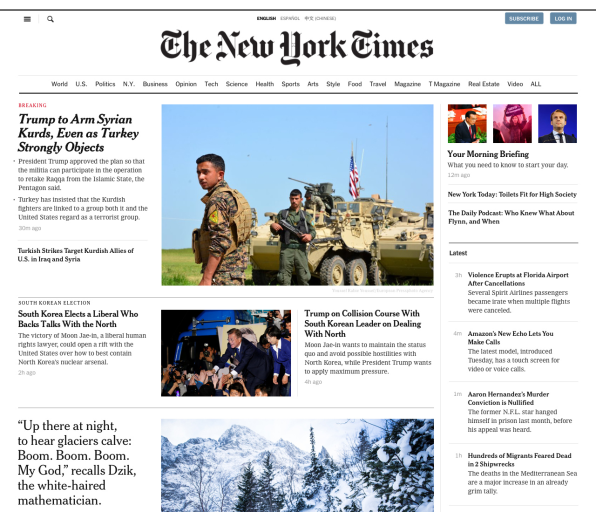In the image, a plethora of headlines and elements are scattered across various parts of the screen, reminiscent of a bustling newsday. 

**Top Right Section**:
- A prominent picture features, where the colors red, purple, and blue stand out distinctly, with a table visible in the background.
- The phrase "Review what you need to know to start your day" is highlighted, suggesting a summary session of vital news points.

**Top Left Section**:
- The header "New York Today" leads, with sub-headers such as "Toilets," "Fairtrade," "Society," "The Daily Mail," and "As I Knew It." A specific mention about Flint places the focus on societal and infrastructural issues.
- Below this header, an image displays soldiers wearing uniforms marked with black on their backs, standing against a background of blue sky and green grass.

**Left Section**:
- Breaking news is prominently featured with the headline "Trump to arm Syrian Kurds even as Turkey strongly objects." This story revolves around President Trump's approval of a plan for the Kurdish militia to participate in the operations to retake Raqqa from the Islamic State. Detailed insights elaborates on Turkey's opposition to Kurdish fighters and the geopolitical tensions involving the U.S., Iraq, Syria, and Kurdish strikes.
- Another significant story covers the South Korean election, declaring the victory of Moon Jae-in, a liberal human rights lawyer. The piece delves into the potential ramifications of his win, particularly concerning U.S.-South Korea relations and North Korea's nuclear arsenal.

**Right Section**:
- A depiction of President Trump appears, suggesting a potential clash with the newly elected South Korean leader, Moon Jae-in, especially regarding strategies to handle North Korea. Moon Jae-in's intention to maintain the status quo is contrasted with the pressure tactics North Korea faces from other international entities.

**Miscellaneous Elements**:
- The taglines "Hamburger Mania," "Magnifying Glass," and a myriad of sections such as "English," "Inscribe," "Plugin," among others, indicate various columns or categories within the publication, ranging from politics, business, opinion, tech, science, to lifestyle and more.
- A disjointed and seemingly surreal narrative mentions individuals, mannequins, and shipwrecks, leading to evocative mentions of actions at an airport after a cancellation, potentially relating to a personal story or societal events.

Overall, this vibrant montage of headlines and images encapsulates a dynamic day in the media landscape, highlighting essential political, societal, and global issues alongside other varied content.